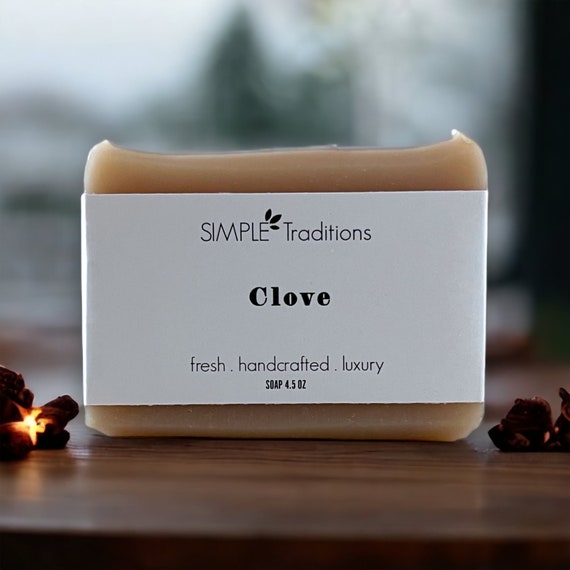The image is a slightly taller than wide square, featuring a bar of soap prominently in the center. The soap is enclosed in a white cardboard sleeve that reads "Simple Traditions, Clove, Fresh Handcrafted Luxury." The text also includes the weight of the soap as 4.5 ounces. The soap itself is a dark beige color, visible at the top and bottom of the packaging. The background showcases a blurred, muted hardwood table, enhancing the focus on the soap. Flanking the soap on both sides are small, darker pieces that appear to be cloves, with one on the left side highlighted by a bright burst of light.